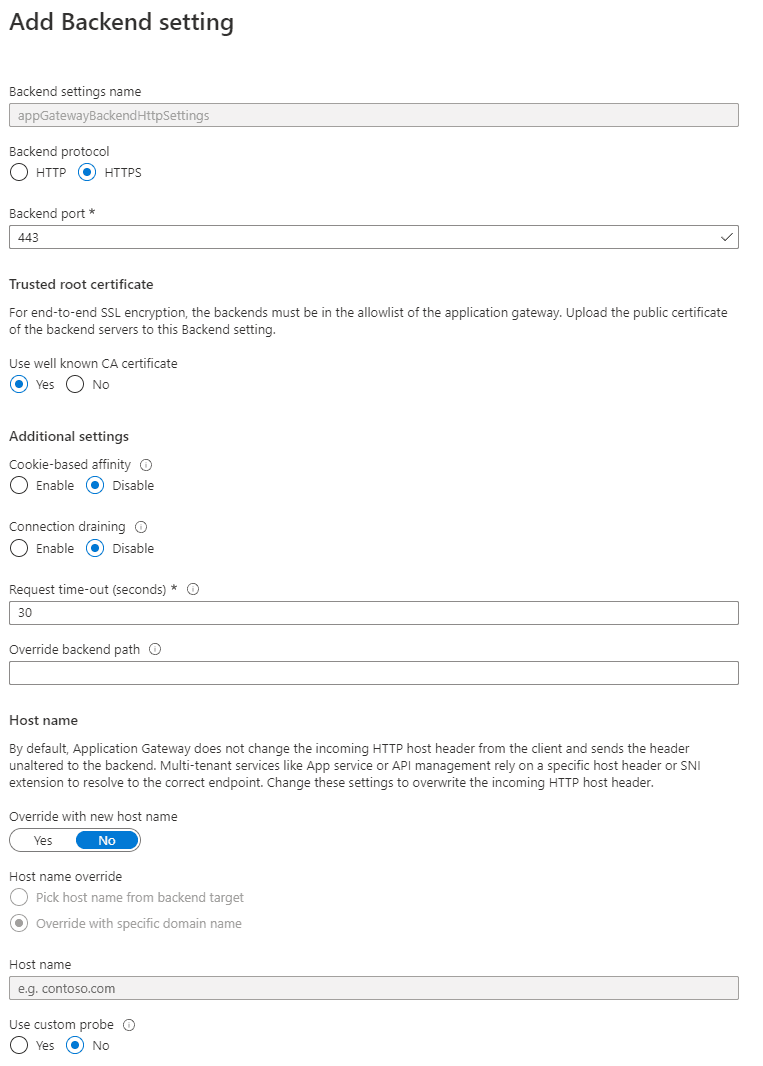The image displays a detailed questionnaire for configuring back-end settings on a website's application gateway. The first question asks for the name of the back-end settings, which has been prefilled as "App Gateway back-end HTTP settings." The chosen back-end protocol is HTTPS, and the required back-end port is set to 443. 

A notification specifies that for end-to-end SSL encryption, the back-end servers must be on the application gateway's allow list. Users are instructed to upload the public certificate of the back-end servers for this back-end setting. The setting for using a well-known CA certificate has been enabled, with the option selected as "Yes."

In the additional settings section, the first option, cookie-based affinity, is set to "Disable." Similarly, connection draining is also set to "Disable." The requested timeout duration is configured to 30 seconds. The host name section indicates that, by default, the application gateway does not alter the incoming HTTP host header from the client; it sends the header unaltered to the back-end.